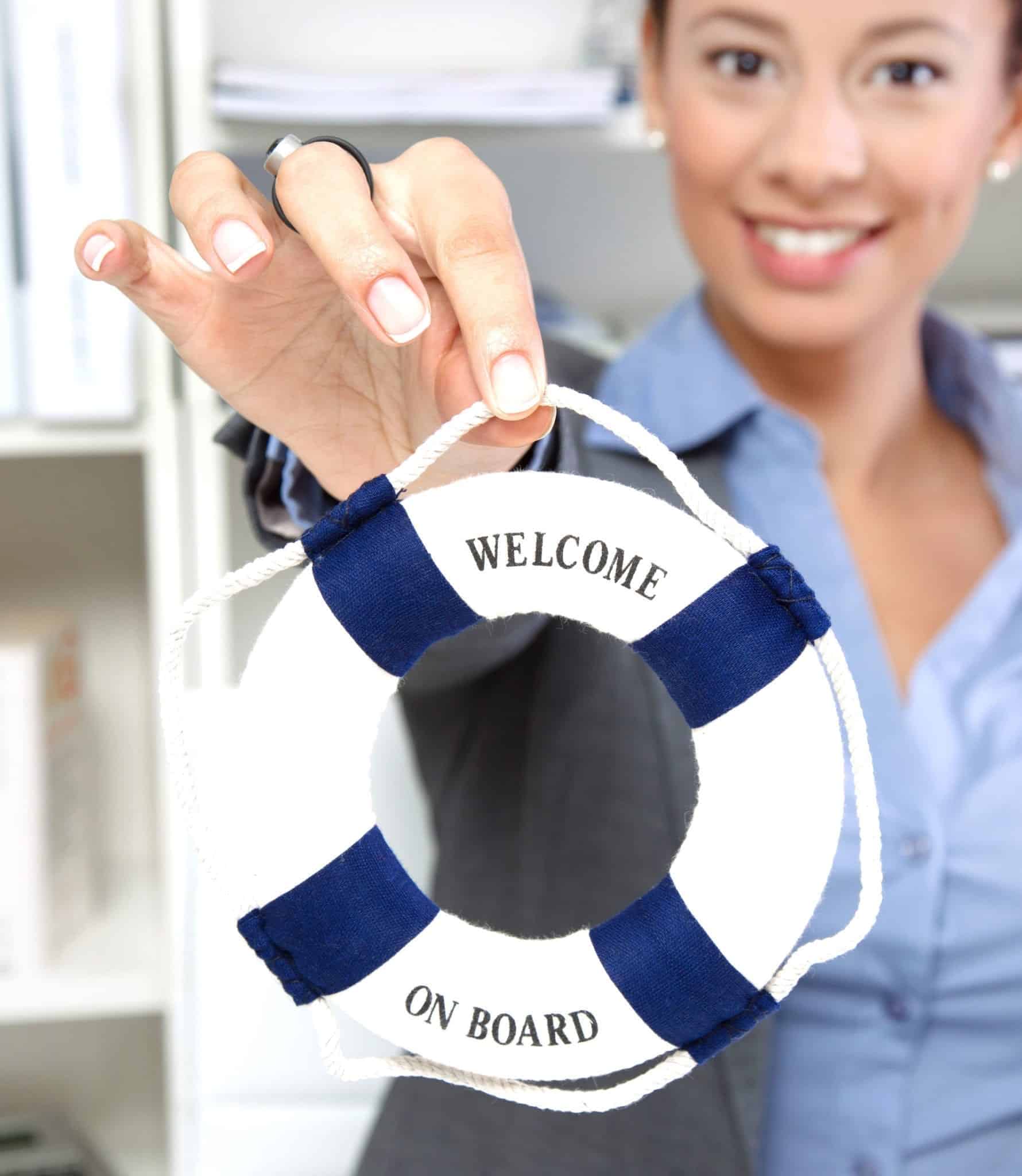A photograph depicts a smiling woman with fair skin and brown eyes, wearing pearl earrings and a black and silver ring on her middle finger, holding out a miniature life preserver. The preserver is circular, white with navy blue fabric accents, and inscribed with "Welcome on Board." Her manicured right hand, pinching the preserver by a string with her thumb and pointer finger, is in sharp focus, while her face and torso are blurred in the background. The woman is donned in a uniform consisting of a light blue collared shirt and a gray jacket, implying she might work on a cruise ship. The colors in the image are muted, featuring shades of white and light blue. Behind her, white shelves filled with binders and various objects add to the backdrop, suggesting an office setting. The muted colors and focus on the life preserver emphasize the central message of welcoming aboard.